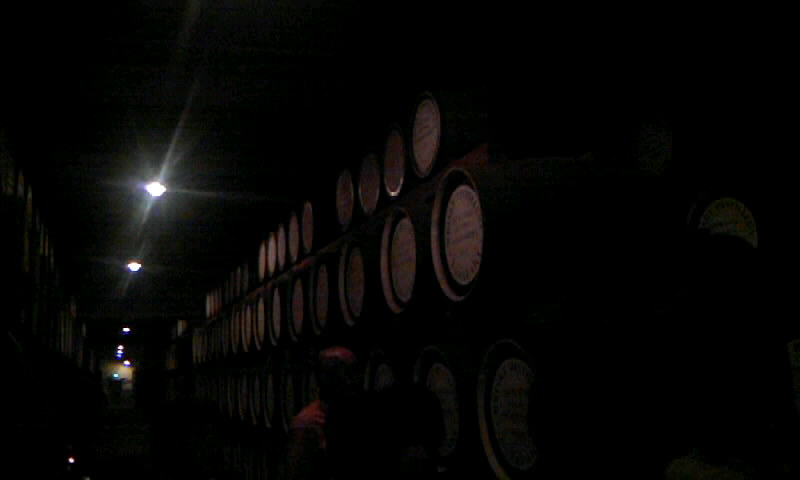The image is an interior shot of a dark, dimly lit storage area within a winery. The photo captures a long, narrow hallway filled with rows of stacked barrels, presumably containing wine. The scene is nearly pitch-black, making it difficult to discern details clearly, but along the left wall, faint white light shines down, revealing small ceiling lights stretching towards the deep background. On the right side, three rows of barrels are visible, each extending from the floor to the ceiling. The ends of these barrels feature large white labels with numerous words and descriptions, though specific text is indistinguishable. Closer to the camera, at the bottom of the frame, the bald head and red shirt of a man are barely noticeable due to the darkness. The hallway’s deep background reveals a room with a softly glowing orange or yellow wall, providing a glimpse of light in an otherwise shadowy scene.